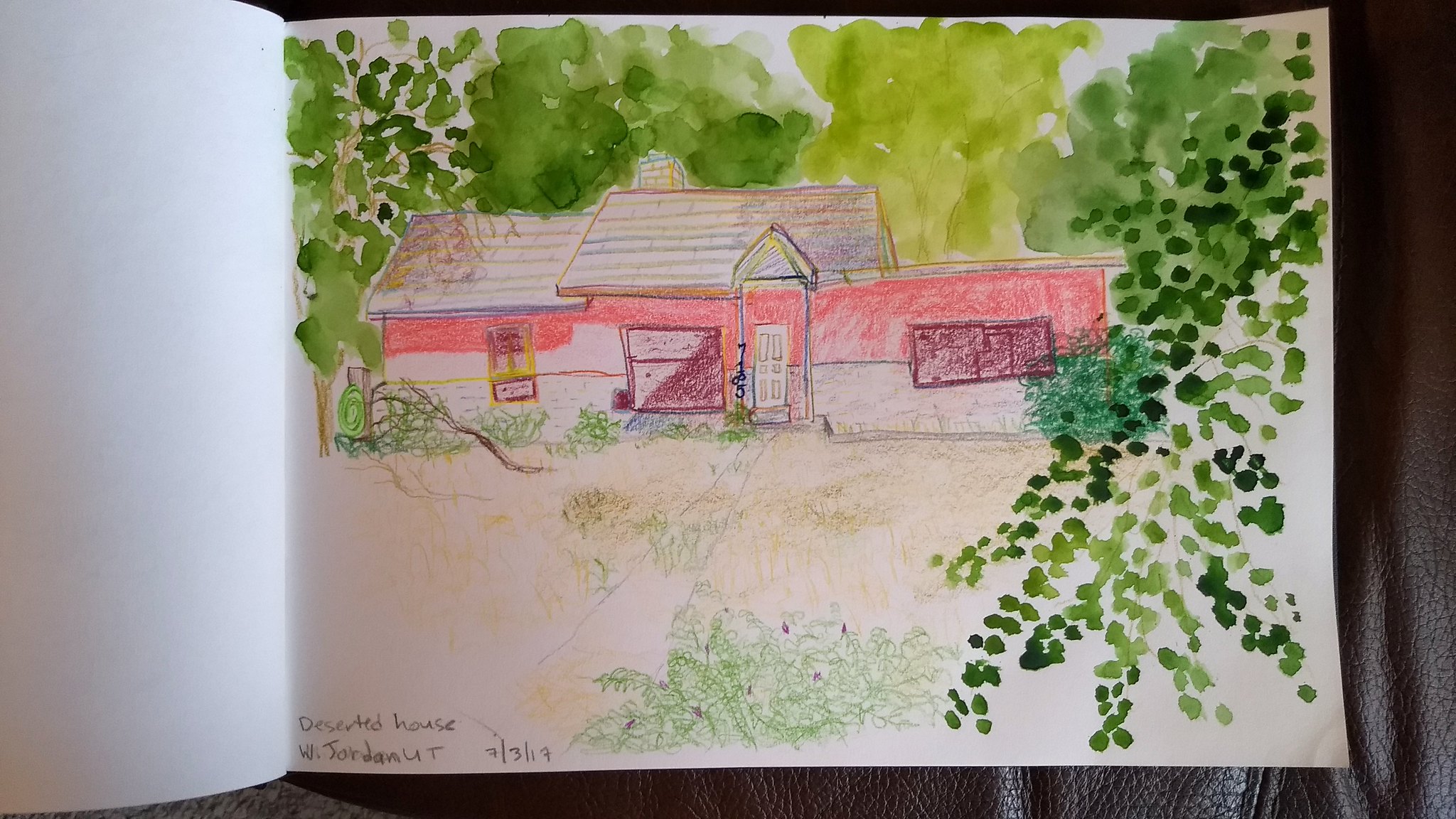This image showcases a childhood drawing of a one-story house credited to "Deserted House, W. Jordan, UT, July 3rd, 2017." The house features a prominent, high-gable entryway with a typical white front door. Flanking the door are two large windows, one on each side, with an additional smaller window to the left. The roof appears to have two levels, complemented by a chimney situated towards the back of the house. Surrounding the house are several trees positioned behind, in front, and to the sides, adding a natural element to the scene. The drawing predominantly showcases an off-white house set against a background of green grass and varied foliage coverage in the front.